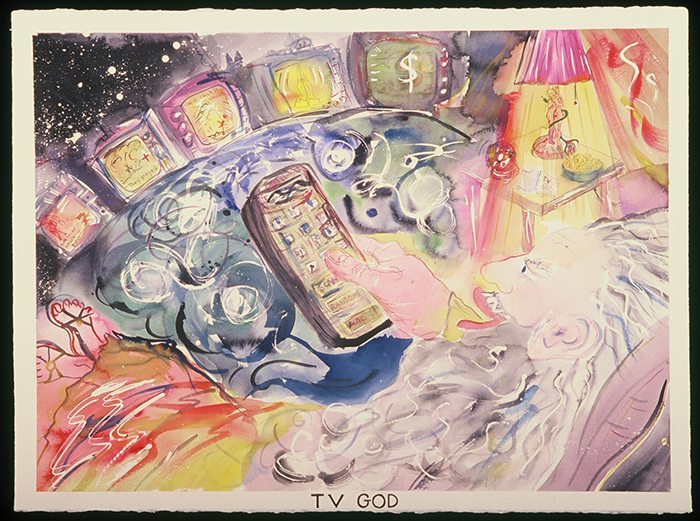This abstract painting, set within a horizontally-oriented, rectangular frame, showcases a multitude of pastel colors and intricate details. The artwork is bordered by an outer black rim frame and an inner beige edge. The central image features a reclining person, seemingly immersed in operating an oversized TV remote control. In front of them are five distinct television screens, set against a black background speckled with white dots that evoke the image of stars.

The person, characterized by their striking red lips and wind-swept hair, is positioned in the lower right corner, settling into a chair. A blue table is situated directly in front of them. To the upper right of the figure, there's a lamp casting a yellow light downward, with the lamp's body intriguingly shaped like a human figure.

The bottom of the painting bears the text “TV guy”, although it was also interpreted as "TV God," adding layers to the possible narrative. Alongside the varied color palette — including shades of black, white, gray, yellow, orange, purple, green, red, and pink — the painting's vivid hues and eclectic mix of household objects create an engaging and visually rich composition suitable for display in a domestic setting.